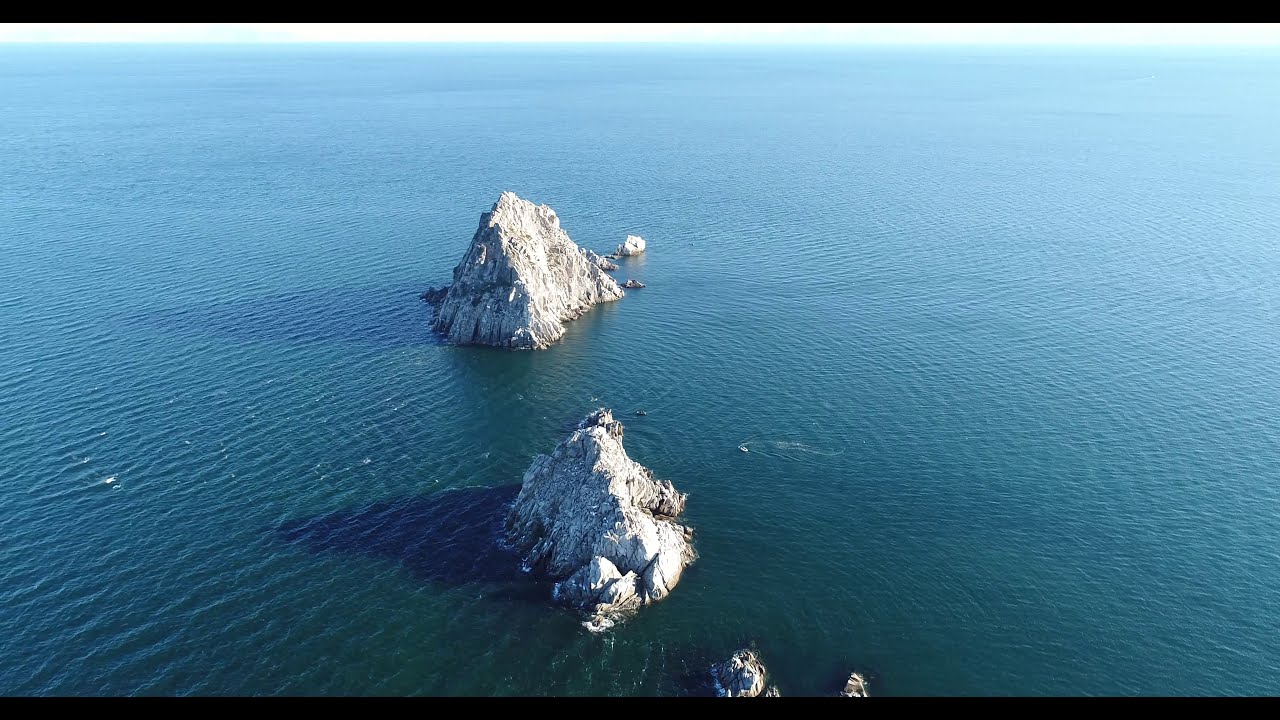The aerial image captures a vast expanse of ocean, extending from the bottom almost to the top, where it meets a thin, bright horizon line under a clear, brightly lit sky. The sunlight is coming from the right side, casting reflections on the left and providing a vivid illumination of the scene. Dominating the bottom center of the image are three steep, stone rock formations that progressively increase in height from the smallest at the bottom to the tallest towards the center. These rocky outcroppings are characterized by their light gray and white pointed tops and curving, sharply sloped sides. Their structures appear jagged and prominent against the rich blue and green hues of the ocean. The water around the rocks ripples gently, emphasizing their stark presence amidst the clear, expansive sea. The entire scene is framed by thin black bars running horizontally along the top and bottom edges of the image, adding a subtle border to the natural beauty on display.